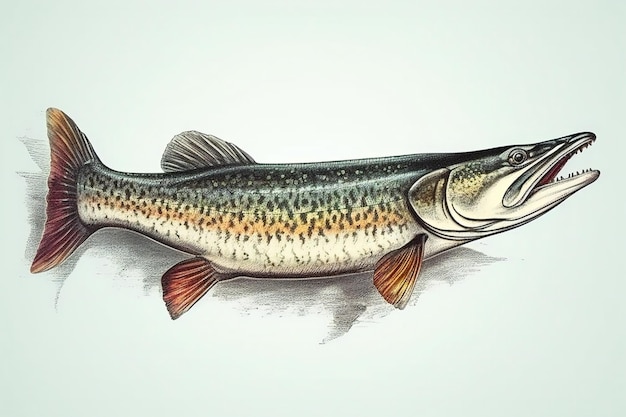The image features a detailed colored pencil illustration of a narrow, vicious-looking fish with its open, fanged mouth pointing to the right. The fish lies flat against a white background with gray, shadowy shading towards the outer corners. The fish, potentially resembling a rainbow trout, displays a complex pattern of black speckles over a series of vivid stripes: the top is black, transitioning to green, then yellow, orange, and finally a white belly, all marked with black speckles. It has an equally colorful tail and fins—orangish-red bottom fins, a top fin in black, and a tail fin in a bright orangish red. The fish’s fierce appearance and the botanical drawing style evoke the works of Audubon or classic anatomical illustrations, emphasizing both its beauty and menacing features.